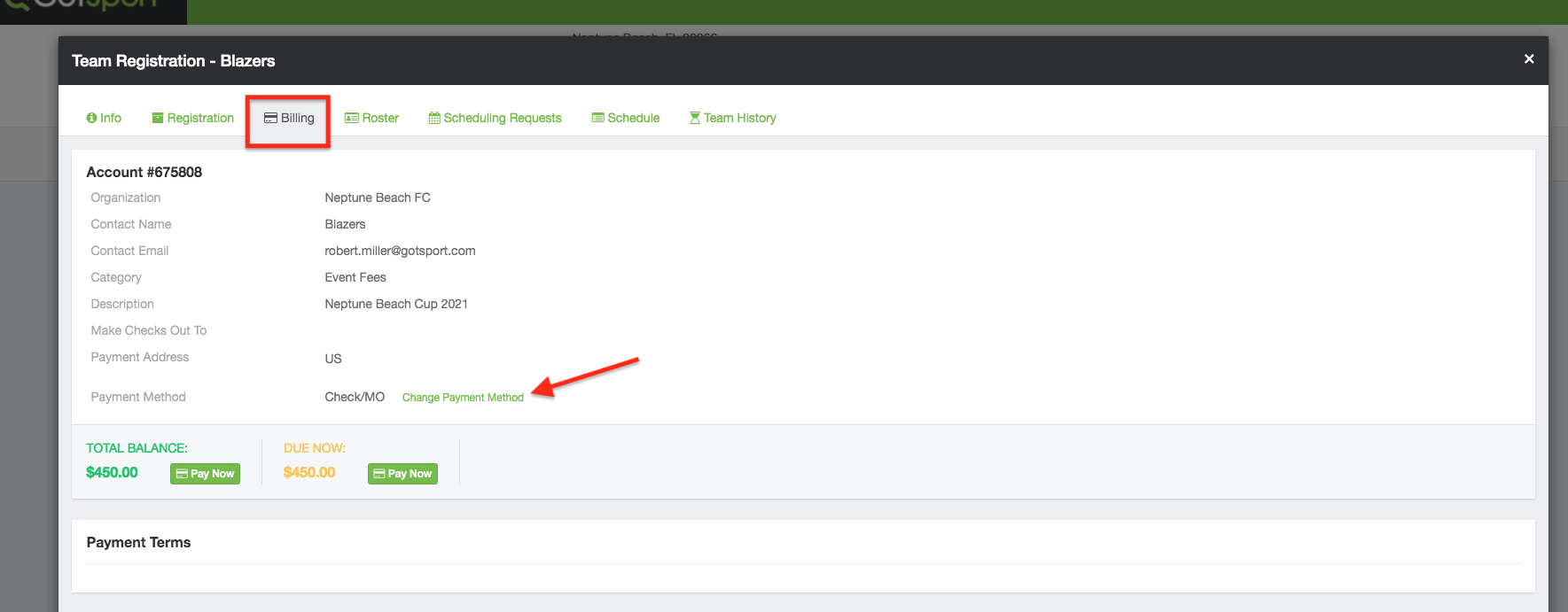In this image, we notice a dashboard for "TeamRegistration - Blazers" prominently displayed at the top left. Below this heading, there are several navigational tabs: Info, Registration, Billing, Roster, Scheduling Requests, Schedule, and Team History. All tabs except for "Billing" are adorned with a green texture; "Billing" is grayed out, indicating it is the currently selected tab, and it is highlighted by a red box.

The section below the tabs is titled "Account" in bold, black text. This section lists detailed information under specific headings: Organization, Contact Name, Contact Email, Category, Payment Address, and Payment Method. Corresponding to these headings, the respective details provided include: Organization as "Beach PG," Name as "Barrera," and Category as "Event Pass."

In the lower left part of the image, there is a boxed area labeled "Total Balance," displaying the amount "450" beside a green "Pay Now" button. Adjacent to this, another boxed area titled "Due Now" (possibly intended as "Out Now") similarly shows the amount "450," though it includes an additional box to the right of the text.